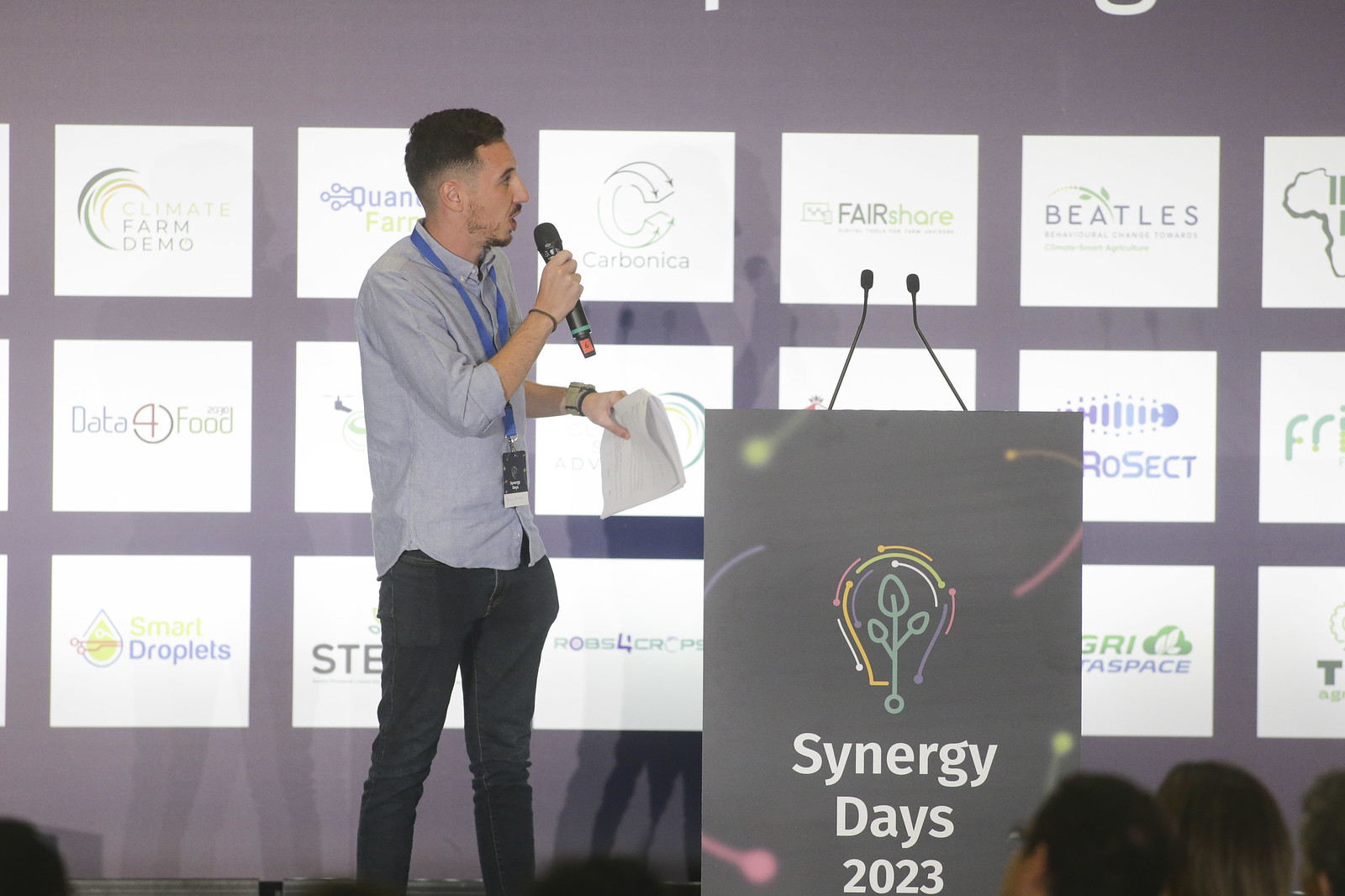The image depicts a scene from Synergy Days 2023, a tech industry conference. At the forefront is a podium adorned with the "Synergy Days 2023" logo, featuring two small microphones. A presenter with short, faded black hair paces back and forth, holding a microphone in his right hand and notes in his left. He is dressed in dark jeans and a light-colored button-up shirt with a bluish lanyard hanging around his neck. In the background, a presentation screen displays several square logos, including those of sponsors like Beatles, Fair Share, and Carbononic. The heads of several attendees are visible at the bottom of the frame, attentively watching the presentation.